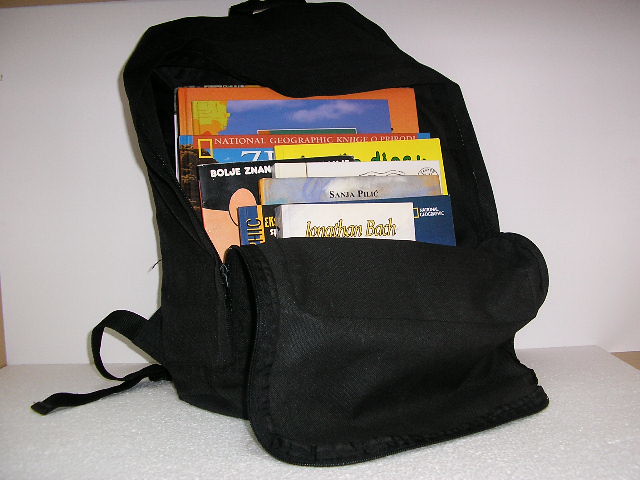A photograph features a black backpack positioned on a white table against a white wall, with a glimpse of a beige floor at the edge of the image. The backpack is fully unzipped, revealing a collection of books within. The front flap of the bag is folded down, exposing the book covers, which overlap each other. Among the visible books, there's a National Geographic book and another with the name "Jonathan Bach" written in yellow with a black outline. The books are of varying colors, including red, blue, yellow, and pink. Behind the backpack, one of the straps is slightly protruding to the side. The white table supports the backpack, though no additional objects or details of the surrounding area are visible.